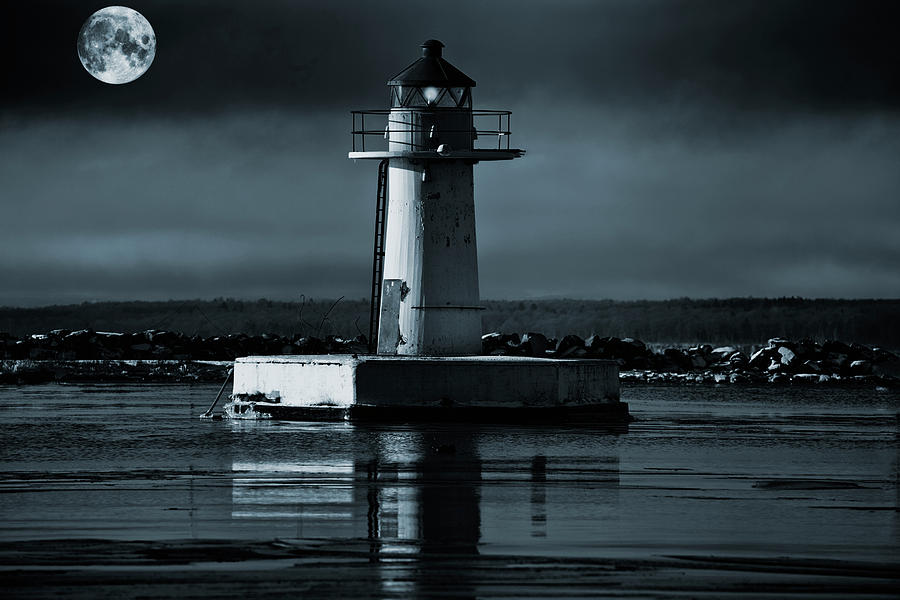The image showcases a serene night-time landscape that blends the realism of a photograph with an uncanny, hyper-realistic or AI-generated quality. Dominating the top left of the image is an incredibly detailed full moon, its surface marked with dark patches and glowing luminescence. The sky, spanning the top third of the frame, is overcast with layered clouds and mist, punctuated by a dark black band near the top. Below, the foreground features a still, reflective body of water that mirrors the scene. 

Central to this composition is a petite, white lighthouse standing on a concrete platform. The lighthouse, distinguished by its cylindrical structure and a subtle black entry door on the left, also has a ladder leading to a circular platform with a railing that encircles its top. The structure is capped with a roof that resembles a conical hat, housing an illuminated white bulb. Just behind the lighthouse, a rocky embankment merges into a narrow strip of land cloaked in shadow. The overall palette is a blend of dark, gray, bluish, and white tones, contributing to its moody, postcard-like aesthetic.